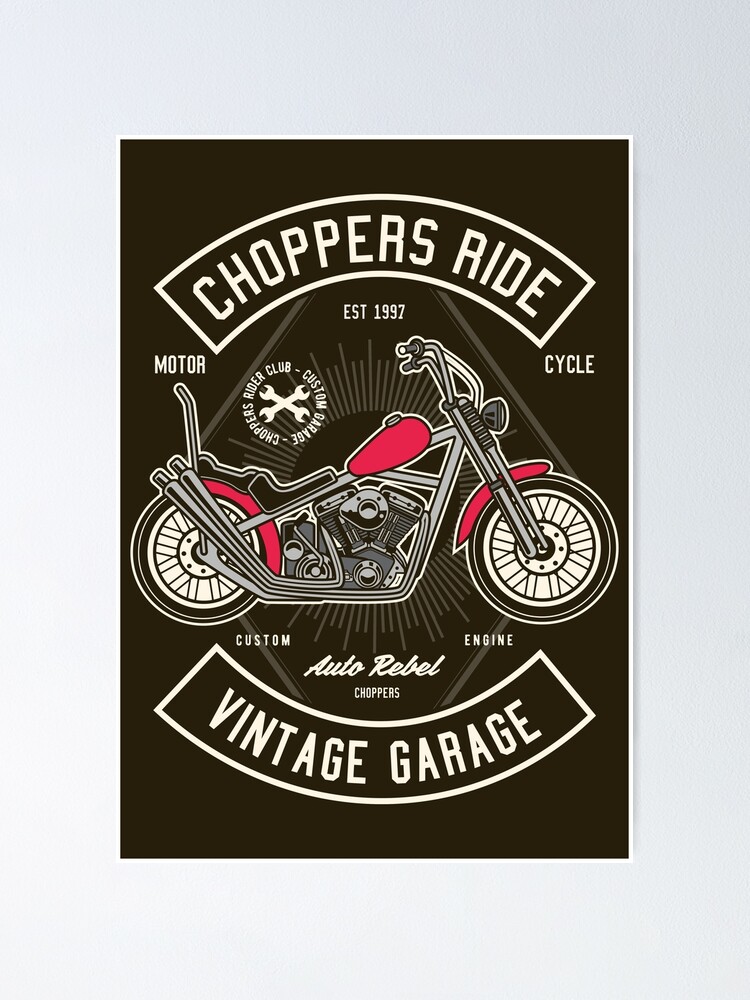Poster Caption:

"Chopper's Ride: Vintage Garage"
At the top of the poster, bold letters read "Chopper's Ride." Directly below, smaller text has the words "Motor" (on the left) and "Cycle" (on the right), with "EST 1997" positioned centrally between them. Beneath this, "Chopper's Rider Club Custom Garage" is prominently displayed.

The focal point of the poster is a cartoon illustration of a red motorcycle shown in a side profile, with its front facing the right and the back facing the left. Underneath the motorcycle image, the text reads "Custom Engine" and "Auto Rebel Choppers."

The background of the poster is black, which makes the artwork and text pop. The entire poster is framed with a gray border, providing a sleek and classic finish.